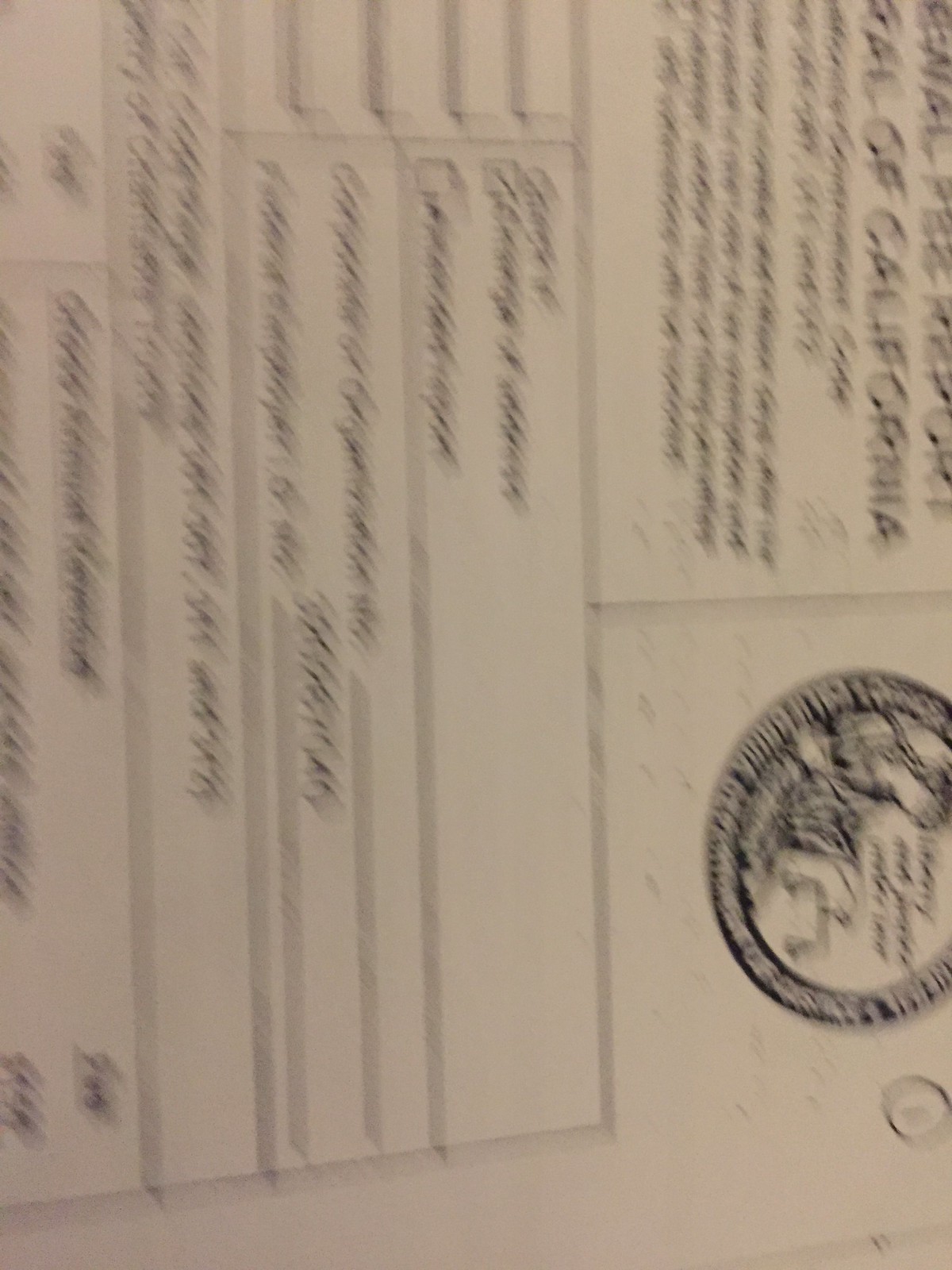This image, though blurry and of low resolution, appears to depict a white sheet of paper positioned sideways. The paper includes various elements, primarily black text, scattered across its surface. Notably, on the bottom right corner, there is a circled number "1" alongside a large, round logo. The overall quality of the image makes it difficult to discern the detailed content of the text and logo, but the primary layout and key elements can be observed.